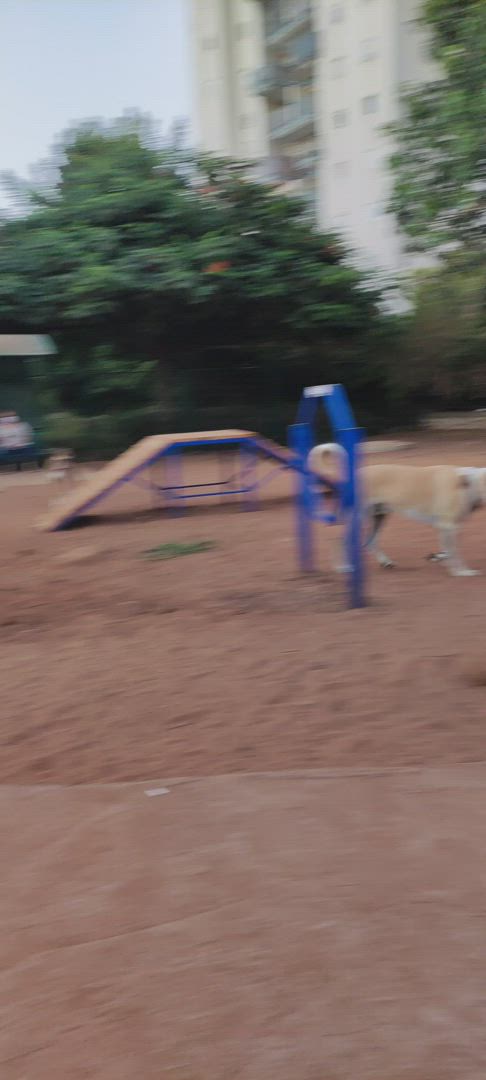In the image, there is a landscape dominated by a vast expanse of dirt, with an engineered ramp structure rising from the ground. This ramp has flat top and blue-colored sides, descending gently on the opposite end. Nestled in the dirt, there is an arched formation. A dog with white fur, possibly tinged with yellow, stands proudly in the foreground, showcasing its curvy tail and white paws. The scene is set against a backdrop of lush green trees and a cloudy, gray sky. Additionally, a tall building with prominent balconies and multiple windows looms in the background, adding an urban contrast to the natural and constructed elements of the image.